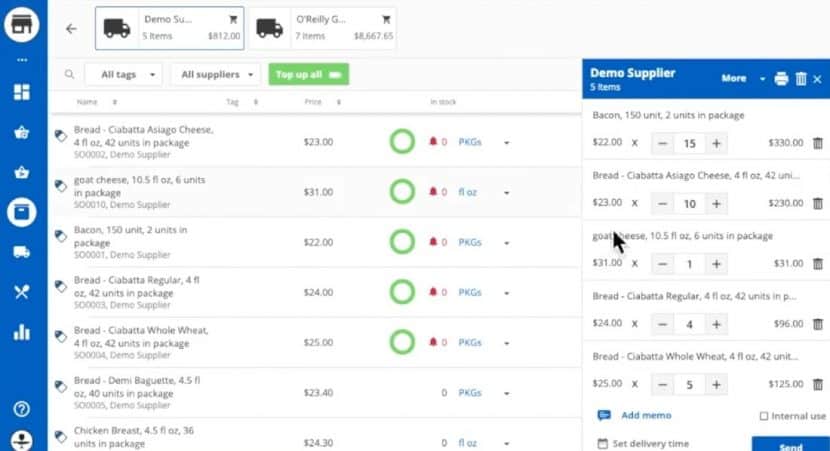Here is a detailed and cleaned-up caption for the image:

---

A screenshot of a website interface showcasing the navigation and main content areas. On the left side of the screen, a vertical blue bar acts as the main menu, featuring seven options. The third option from the top is highlighted, indicated by a white circle surrounding a blue icon, distinguishing it from other white icons. At the top-right corner, the word "Demo" is prominently displayed next to initials "SU" encased in a grey rectangle, suggesting a demo mode or user profile. Below this, another rectangle displays a truck icon and the label "O'Reilly G." Below that, filters for "All Tags" and "All Suppliers" are present. The main content area lists items such as bread, goat cheese, and bacon, likely representing a product or inventory list.